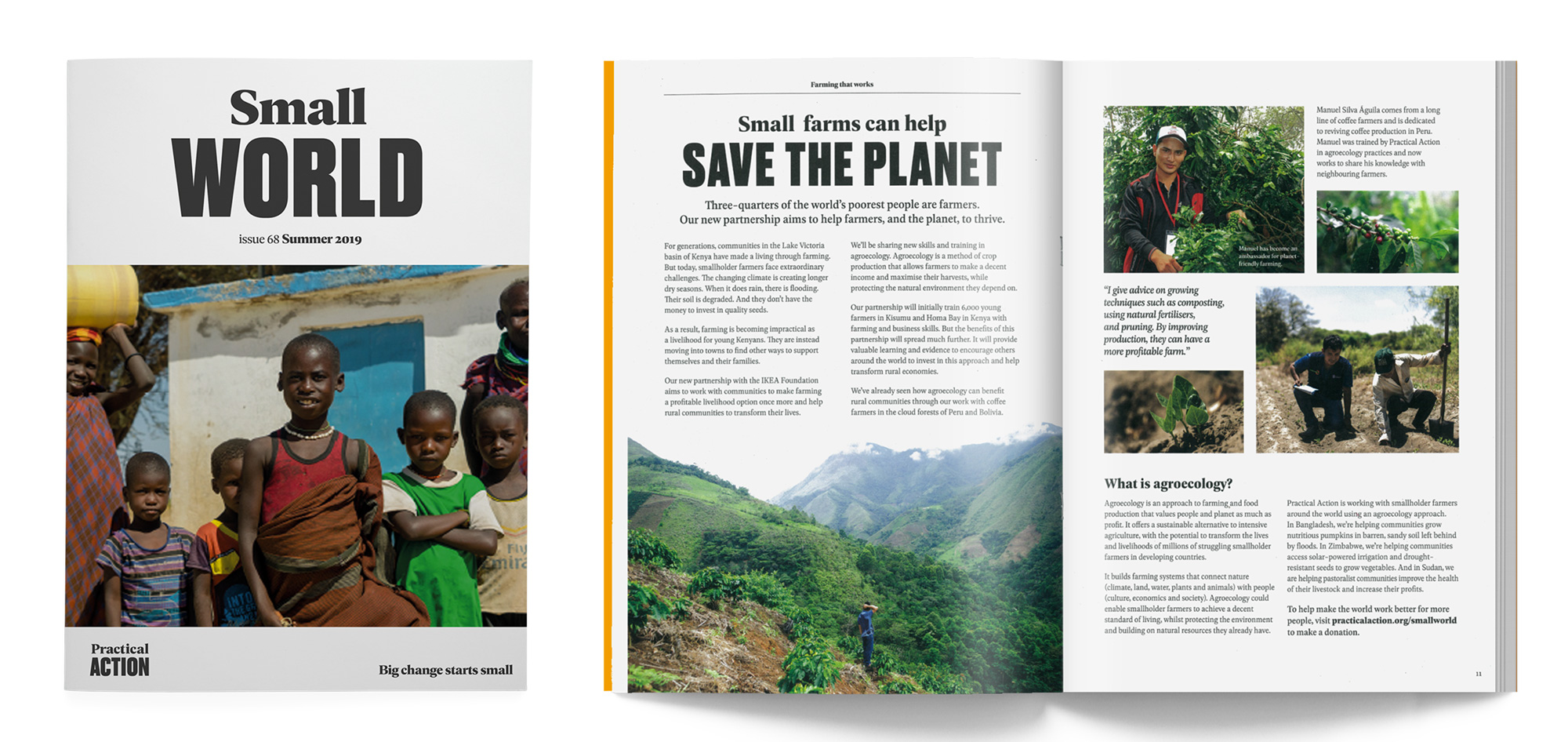The image comprises a detailed screenshot of a magazine cover accompanied by an interior glimpse of an article within the issue. Here's the cleaned-up and detailed descriptive caption:

---

The image features the cover of a magazine titled "Small World." The cover utilizes a minimalist design with grey bands at the top and bottom, and prominently displayed, large black text in the center that reads "Small World." Subtitled in smaller black text, it states "Issue 68, Summer 2019." Central to the cover is a striking photograph depicting a group of African children looking directly at the camera. Though most have serious expressions, the child at the center and one on the left side are subtly smiling. The children are dressed in vibrant clothing in shades of red, green, blue, yellow, and white. In the bottom left corner of the cover, the text "Practical Action" is visible, while the phrase "Big change starts small" is inscribed on the right-hand side.

Accompanying the cover image is another photograph showcasing an open spread from the magazine. The top of this page has some unreadable black text above a thin red bar. A vertical yellow bar runs down the left side of the spread. Returning to the first page, prominent black text in the middle of the left page reads "Small farms can save the planet," accompanied by a dense block of text underneath. Below this, a picturesque image of verdant hills dominates the lower part of the page. On the right-hand page, there are four smaller images arranged vertically, depicting people engaged in agricultural activities. The headline "What is Agroecology?" appears, followed by extensive explanatory black text, probably detailing the content and relevance of the accompanying images and the agricultural theme of the article.

---